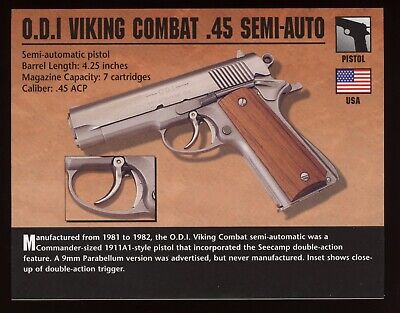The image is an advertisement for a handgun titled "O.D.I. Viking Combat .45 Semi-Auto." The central illustration, akin to those found in magazines, features a detailed drawing of the gun on a brown-tan background bordered in black. The handgun is depicted with a silver finish and a wooden handle, and there's a zoomed-in detail of the double-action trigger on the side. 

At the top, specifications are listed: "O.D.I. Viking Combat .45 Semi-Automatic Pistol, Barrel Length 4.25 inches, Magazine Capacity 7 Cartridges, Caliber .45 ACP.” The upper right corner hosts a gray logo that reads "pistol" with an image of the U.S. flag and the text "USA" beneath it.

The bottom of the advertisement includes a black-bordered informational section stating, "Manufactured from 1981 to 1982, the O.D.I. Viking Combat Semi-Automatic was a commander-sized 1911A1 style pistol that incorporated the C-Camp double-action feature. A 9mm Parabellum version was advertised but never manufactured. The inset shows a close-up of the double-action trigger."